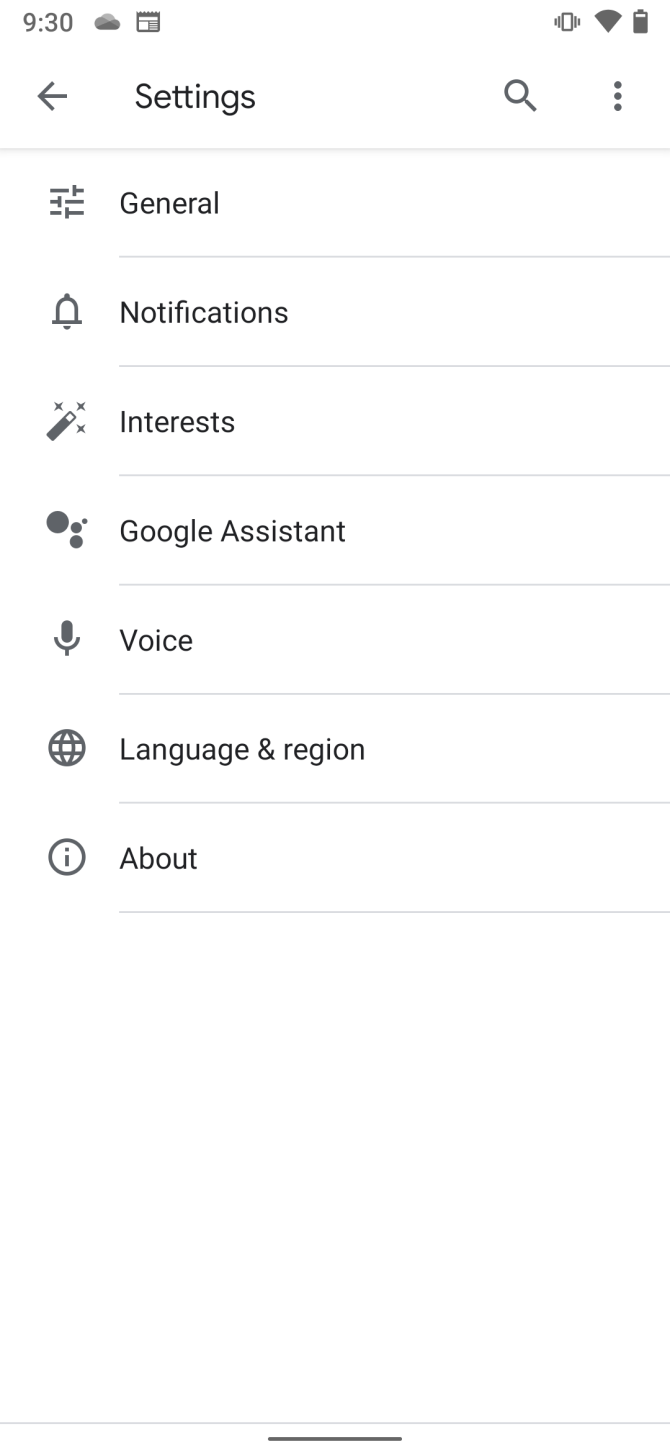At the top left corner of the image, the time is displayed as 9:30. Next to the time, there is a small cloud icon followed by a notebook icon. An arrow pointing to the left is located beside the word “Settings,” and adjacent to it is a magnifying glass icon symbolizing the search function.

Beneath this header area, various menu items are listed in a structured format, each separated by thin gray horizontal lines. The first item has three lines next to it and is labeled "General." The next item features a bell icon with the word "Notifications." Following this, there's an icon resembling a magic wand surrounded by stars and the word "Interests."

Further down, a circle icon is displayed alongside a smaller circle, next to which is the label "Google Assistant." Subsequent to this is a microphone icon with the word "Voice" spelled out as V-O-I-C-E. Then, an icon of a globe is present with the label "Language and Region" in black text.

Lastly, there is a circle containing a lowercase "i," next to which the word "About" is written.

In the upper right corner of the image, the icon of a nearly fully charged cell phone battery is visible.